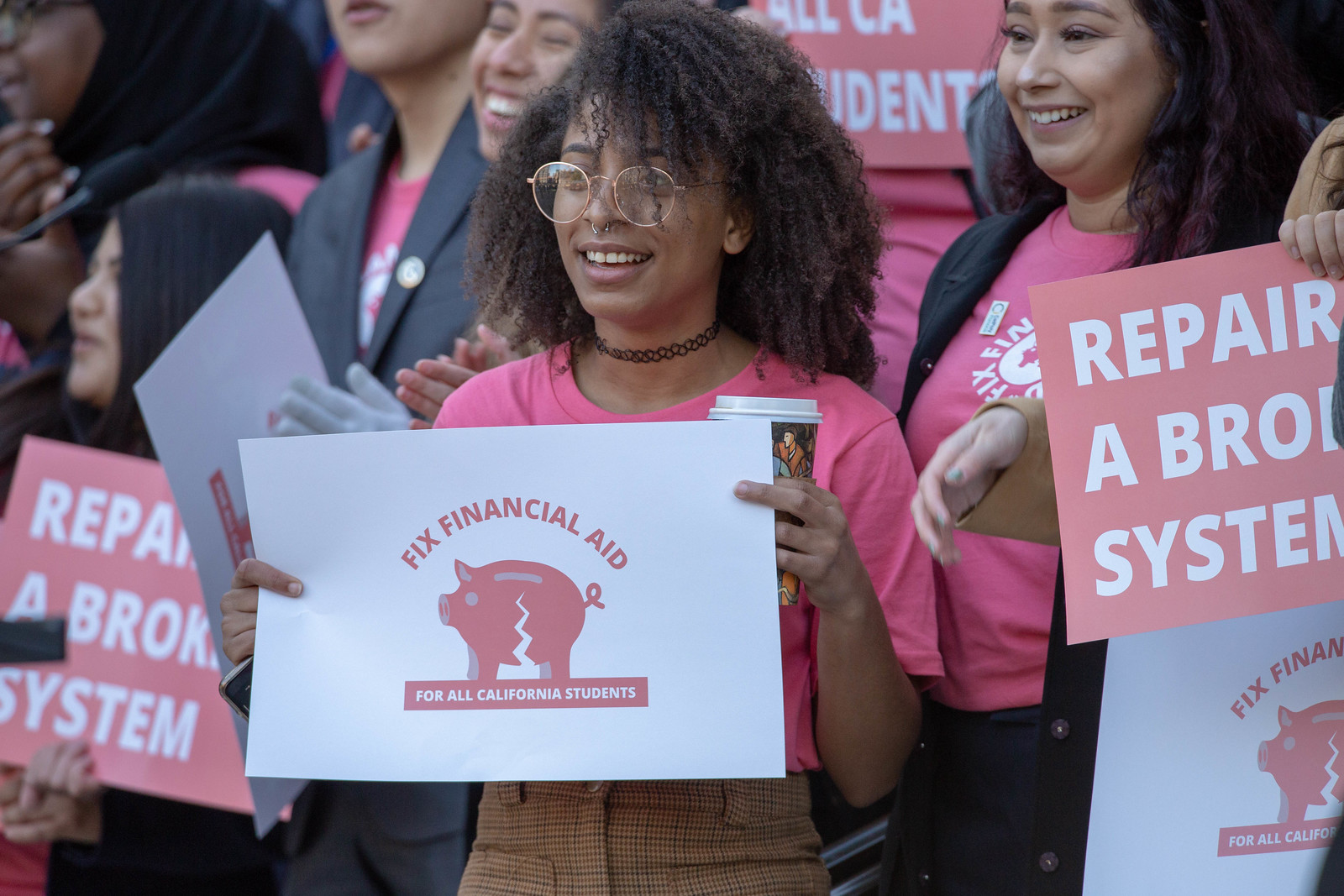In this wide rectangular image, a group of women, seemingly students in California, are peacefully protesting issues with the financial aid system. All the women, about six or seven in total, are wearing pink short-sleeve shirts, which appear to signify their unity and cause. The focal point of the image is a light-skinned woman at the center, slightly tilted diagonally to the left. She is smiling, with her curly brown hair cascading around her thin-rimmed glasses, and she has a silver nose piercing. She is dressed in brown plaid pants and holds a cup of coffee in her left hand while holding a white rectangular sign in both hands that reads, "Fix Financial Aid." The sign features a picture of a broken piggy bank and the additional text, "For All California Students."

To her right, another woman with darker, wavier hair, and light brown skin can be seen laughing. She is wearing a dark blazer over her pink shirt and dark pants. Other women in the background are also holding signs, many of which carry messages about repairing the financial aid system. The image captures a combination of determination and camaraderie among the protesters, showcasing their collective call to action for financial reform in a spirited yet peaceful manner.